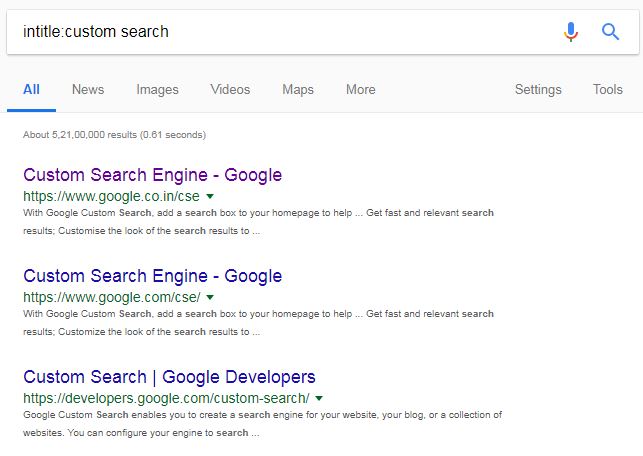The image is a screenshot of a Google search engine results page. The background at the very top is white. Prominently displayed is the search box, a long white rectangle, with text inside that reads "custom search." To the left of the search box, the title "Custom Search" is written in clean blue font. On the right side, there are two icons: a gray microphone (enabling voice search) and a blue circle with a magnifying glass icon (used for initiating the search).

Below the search box, there are navigational categories, with "All" highlighted in blue, indicating it's the selected tab. The other categories, displayed in gray, are "News," "Images," "Videos," "Maps," "More," "Settings," and "Tools," showing the various filter options available.

Immediately beneath these categories, the page indicates the search results: "About 5,021,100,000 results (0.61 seconds)." Following this information, several search result entries are listed.

The first result is titled "Custom Search Engine - Google" with the web address "https://www.co.in/cse." The second result also reads "Custom Search Engine - Google" with a different web address. The third result is titled "Custom Search | Google Developers" and has the web address "https://developers.google.com/custom-search/." Each entry appears standardized, indicating different resources related to Google's custom search engine.